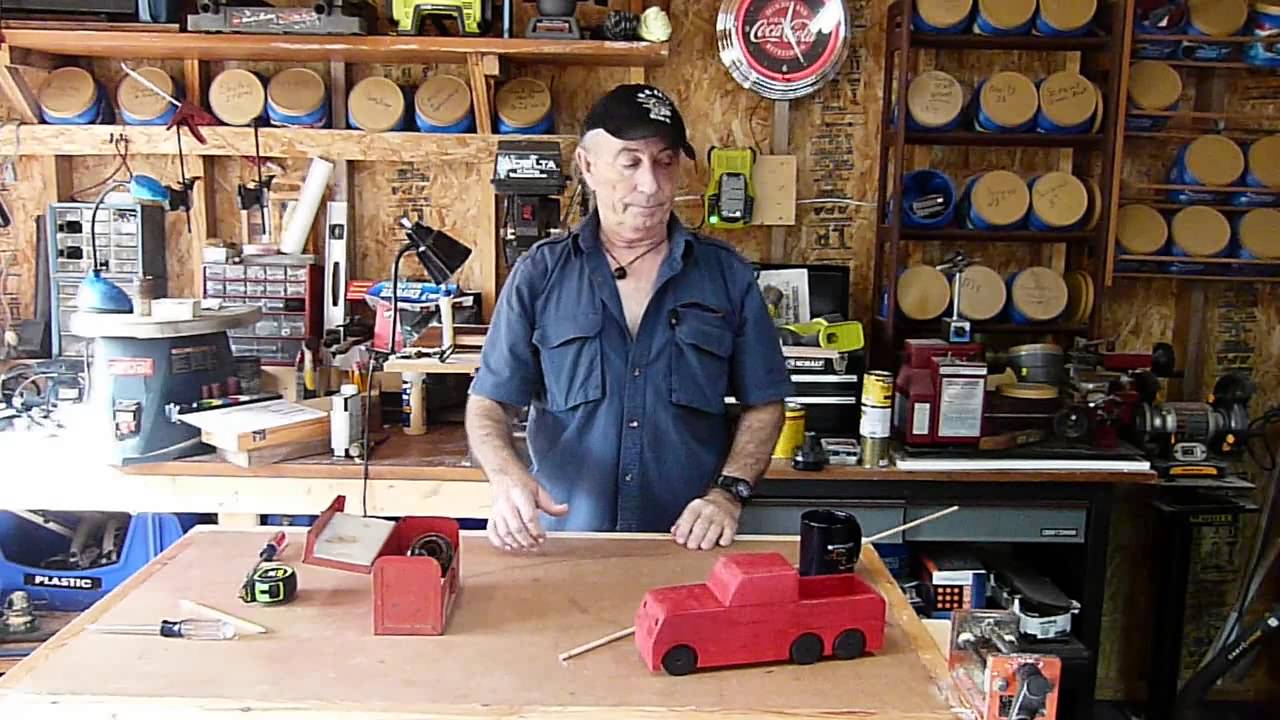In this casual image, a man who appears to be in his 60s is captured unaware in his workshop. He is wearing a short-sleeve, dark blue button-down shirt with two chest pockets, a black wristwatch, and a black baseball cap, and is standing beside a square wooden work table. On the table, there is a red-painted wooden toy truck with little black wheels, a black coffee mug, a clear screwdriver, and a red toolbox with a black object inside. The background showcases raw plywood walls adorned with various tools and equipment, including shelves brimming with jars and canisters that have handwritten black labels. Above him, a circular Coca-Cola clock with a silver border indicates it's midday. The workspace is filled with an assortment of items like screws, nails, and other handyman essentials, alongside a black lamp providing light. The overall setting is rich in earthy browns, creating a warm, busy atmosphere characteristic of a well-used workshop.